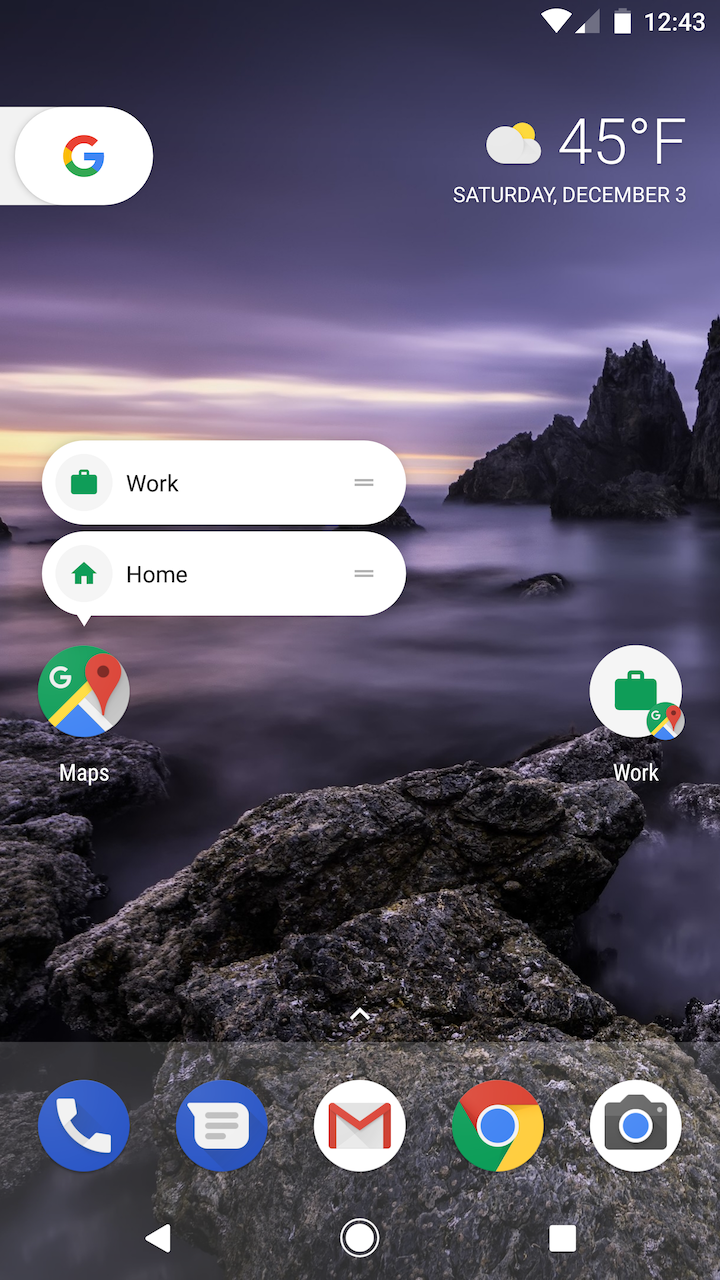This image is a detailed screenshot of a smartphone home screen. At the top right corner, the time displayed is 12:43, and next to it are various icons. The battery icon shows approximately 90% charge, the cellular signal icon appears to be at about 30% strength, and the Wi-Fi signal icon is a solid triangle with a rounded top.

The phone's wallpaper is a stunning landscape photo depicting a rocky coastline. Dark rocks occupy both the foreground and background, with some taller formations jutting out from what seems to be a misty or foggy area near the water's edge. In the distance, the golden hues of a sunset can be seen, transitioning to light purple clouds accented with more golden tones, eventually darkening into a grayish purple higher up.

Directly under the time on the top right corner is a small weather icon showing a cloud with the sun peeking from behind, accompanied by the temperature, 45 degrees Fahrenheit. On the opposite corner, the top left, is a Google icon, and next to it is a slide button.

Midway down the screen, there are Google Maps shortcuts represented by a circular icon. Above it are two chat box icons labeled "Home" and "Work". The "Home" icon is white with a small house symbol to the left and two gray menu lines to the right. The "Work" icon is green with a briefcase symbol to the left and similar gray menu lines to the right. There's another shortcut in the bottom right corner featuring a round icon with a green briefcase inside it, adjacent to a small white round Maps icon.

At the very bottom of the screen, five circular icons are displayed from left to right: a phone icon, a text message chat bubble with a blue background, a Gmail icon showing a red and white envelope, the Chrome browser icon with its signature red, yellow, green, and blue colors, and a camera icon with a white background and a black camera symbol. The camera icon includes a white circle and a blue circle in the middle, featuring a small white square underneath. Adjacent to it on the left is a white icon resembling a record button. Further left from that is a white triangle pointing to the left.

This detailed snapshot encompasses various essential features and visually appealing elements of the smartphone's user interface.